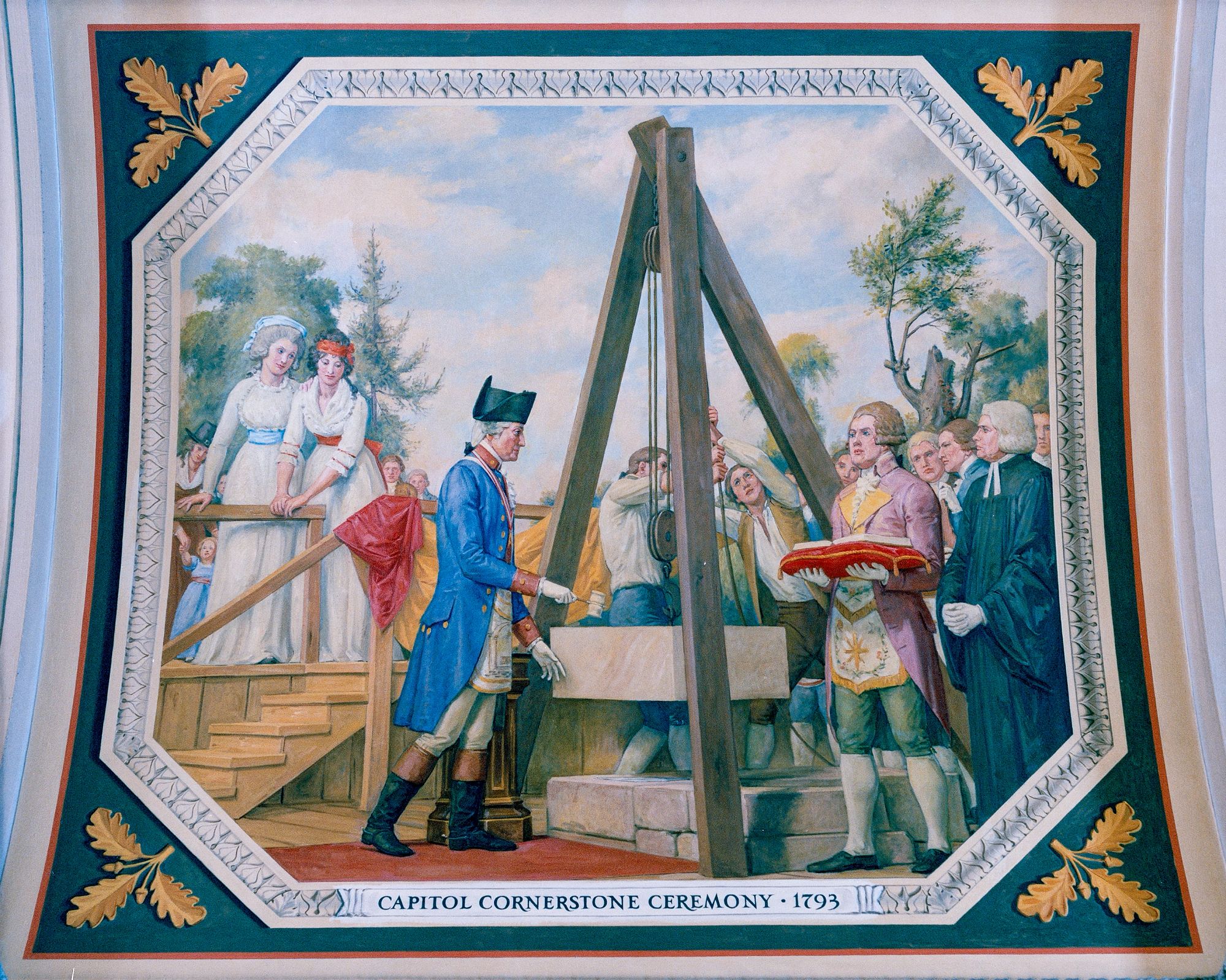The painting depicts an early colonial scene from 1793, titled "Capitol Cornerstone Ceremony." Central to the composition is a well-coordinated group of men and women in period attire. The men are meticulously working together, using ropes and a rig to lift a heavy cornerstone. This stone, labeled "Capitol Cornerstone Ceremony, 1793," signifies the historical importance of the event.

On the right, a man stands holding a red pillow as if presenting something of great significance. Next to him is a distinguished figure wearing a large blue coat, complete with a black hat, white hair, and sunglasses, suggesting his prominence and leadership, possibly a general. To the left of these figures, two women in long white dresses observe the ceremony from a platform with attentive and admiring expressions. The left side also features another man in a military uniform, characterized by a very long coat, tall boots, and a hat.

The scene is framed in a way that highlights the collaborative effort and solemnity of the occasion, encapsulating the historical and social dynamics of early colonial America.